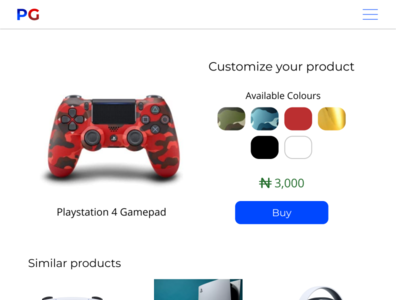The image showcases a clean and straightforward sales page for a PlayStation 4 game pad. Set against a white background, the upper left corner features a blue capital 'P' beside a red capital 'G'. In the top right corner, three blue horizontal lines are stacked one above the other.

Toward the center left, there is a vivid photograph of the game pad itself. The controller is predominantly red, infused with swirling patterns reminiscent of khaki but in red hues. The design is sleek and typical of standard game pads, complete with the usual array of controls. Beneath the image, the text reads, "PlayStation 4 Game Pad."

To the right of the photograph, the text invites users to "Customize your product." It lists five available colors, spelled in British English as "Colours." The color choices include khaki, blue khaki, red, gold, black, and white.

Positioned below this customization section is the price, denoted with an 'N' symbol featuring two horizontal lines, suggesting a stylized currency indicator. The stated price is $3,000. A blue rectangular button beneath the price bears the word "Buy" in white text.

At the bottom left of the page, there is a section labeled "Similar Products," which displays three additional product images. However, only the tops of these images are visible as the page ends abruptly.

Overall, the design is minimalistic, focusing on the essential details and the vibrant image of the game pad to attract potential buyers.